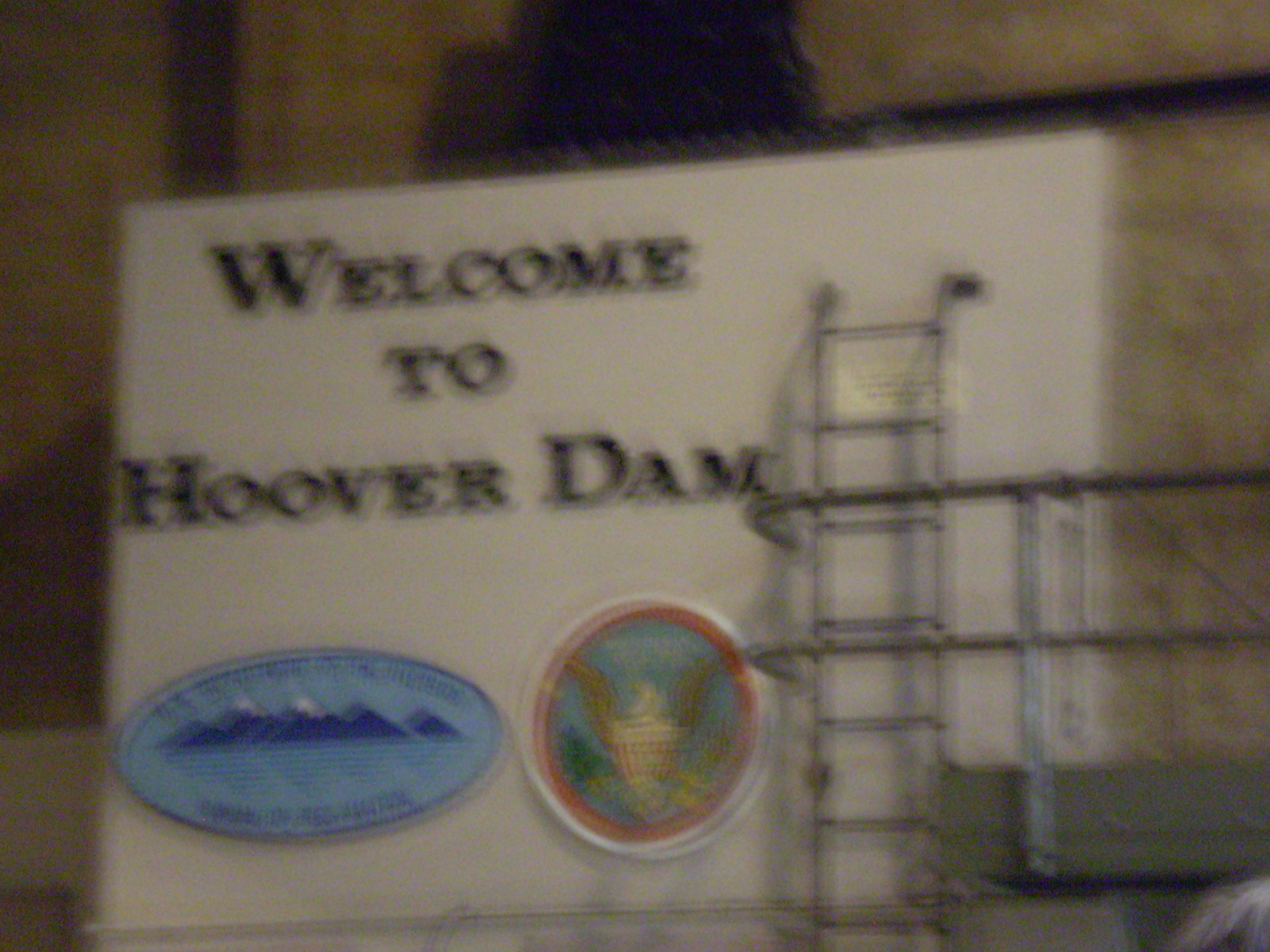This colour photograph, though quite blurred and dark as if taken at night or underexposed, prominently features a large sign occupying the center 80% of the frame. The sign appears greyish, though it may actually be white, with black lettering that reads "Welcome to Hoover Dam." Below this, to the left, is a blue horizontal oval logo depicting an outline of mountains and sea, with some blue writing on the top and bottom. To the right of this oval logo is a round emblem with an orange outer ring, featuring what might be a yellow eagle or crest on a blue background.

Beside these logos, a silver metal ladder is visible, extending nearly to the top of the sign and seemingly attached via small feet. Attached to this ladder near the top is a small yellow sign with black writing. The ladder appears to be behind several horizontal iron bars, which may be part of a cart or trailer, forming the base of the image. The background of the photograph is very dark, with a brownish hue and some indistinguishable shadows in the upper part.